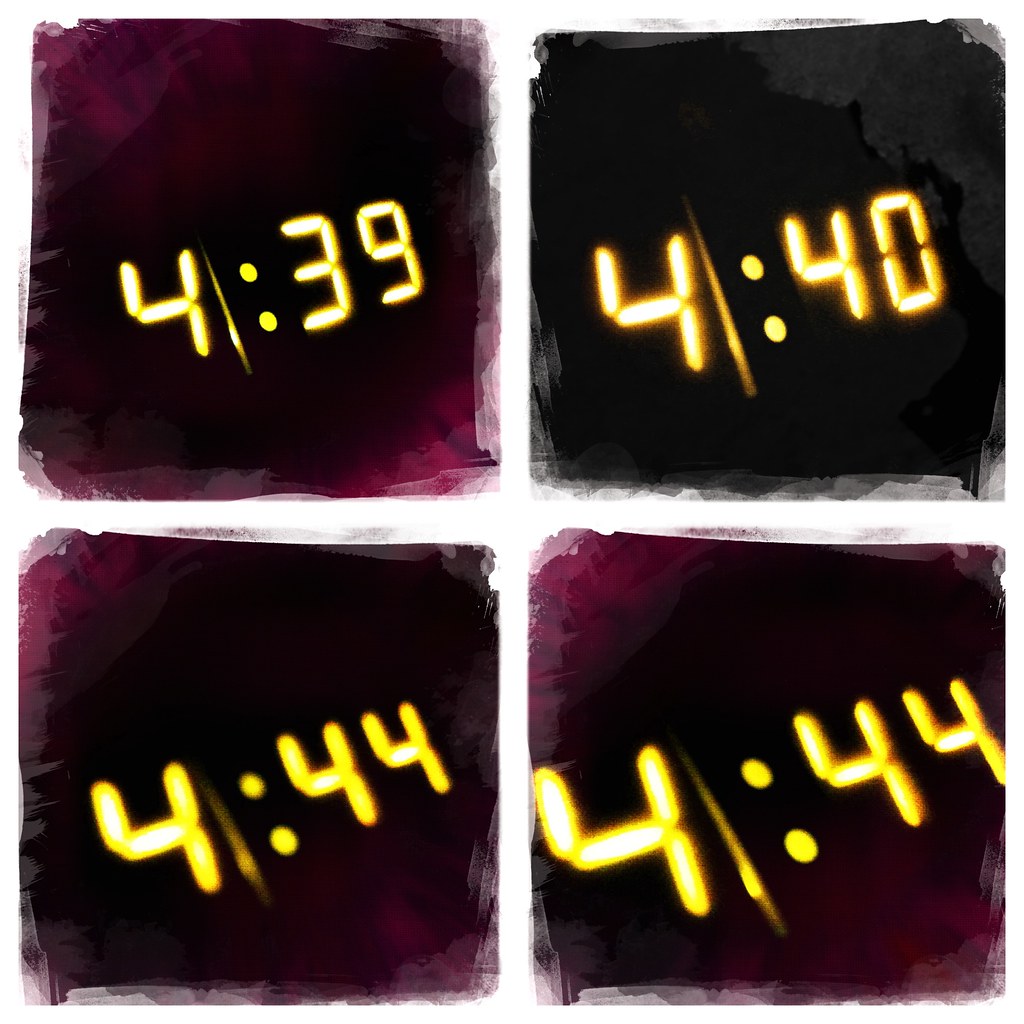The image consists of a grid of four sections, each showcasing a different view of an alarm clock display with distinct times and backgrounds. The top-left quadrant features the time 4:39 with a purplish background that fades to lighter purple towards the edges. The top-right quadrant displays the time 4:40 against a very dark, almost black background. The bottom-left quadrant shows the time 4:44 with a deep cranberry to burgundy background that transitions to lighter shades at the edges. The bottom-right quadrant also displays 4:44, but this image is zoomed in, making the numbers appear larger, and shares a similar burgundy to purplish background. All the times are displayed in bright yellow digits. The backgrounds of each quadrant have a watercolor design, adding a textured and artistic feel to the overall image.